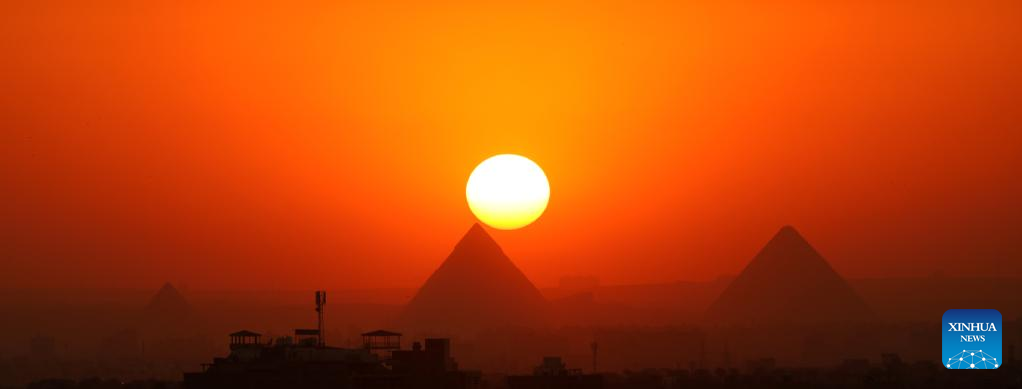A stunning panoramic photograph captures the majestic scene of three Egyptian pyramids with the vibrant, round Sun setting in the background, casting the sky in a hazy gradient of red, orange, and yellow hues. The photograph's outer corners are enveloped in deep red, transitioning to orange and golden tones as they converge around the brilliant Sun near the center. The largest of the pyramids, located centrally, almost touches the Sun with its apex, flanked by a slightly smaller pyramid on the right and a diminutive one on the left, barely cresting the horizon. In the foreground, shadows obscure what seem to be vehicles, likely tourist transports, and several indistinct structures, possibly tents, situated on platforms or hills. The bottom right corner of the image is marked by a blue square logo bearing the text "XINHUA NEWS" in white letters. The overall composition guides the viewer's eye from the vivid sky and radiant Sun to the iconic pyramids, capturing a quintessential yet ethereal view of this ancient landscape.